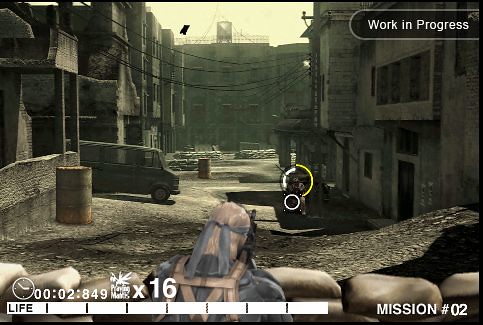In this "Metal Gear" game image, the top right corner prominently displays the text "Work in Progress," indicating that the image is from an unfinished version of the game. The bottom right corner features "Mission Number 0-2," suggesting this is part of a specific mission sequence. On the bottom left, a "Length Bar" is shown, likely representing some form of progress or duration metric. There are multiple white squares depicted, with a clock showing the time as "00:00:28:49."

In the background, a run-down cityscape is visible, characterized by stone walls and gray skies, contributing to a bleak atmosphere. A black truck or van with black wheels is situated in this urban decay. There's an objective marker or goal indicator located in the mid-right area of the screen, suggesting a point of interest or mission target.

In the immediate foreground, the perspective appears to be from a character aiming over some sandbags or barricades. A man with distinctive white hair, a gray bandana, and a brown vest is seen, likely a key character in the scene. Above him, the word "Phantom" appears, along with the name "Mantis" or "Praying Mantis" repeated 16 times, which could refer to a specific enemy or element within the game.